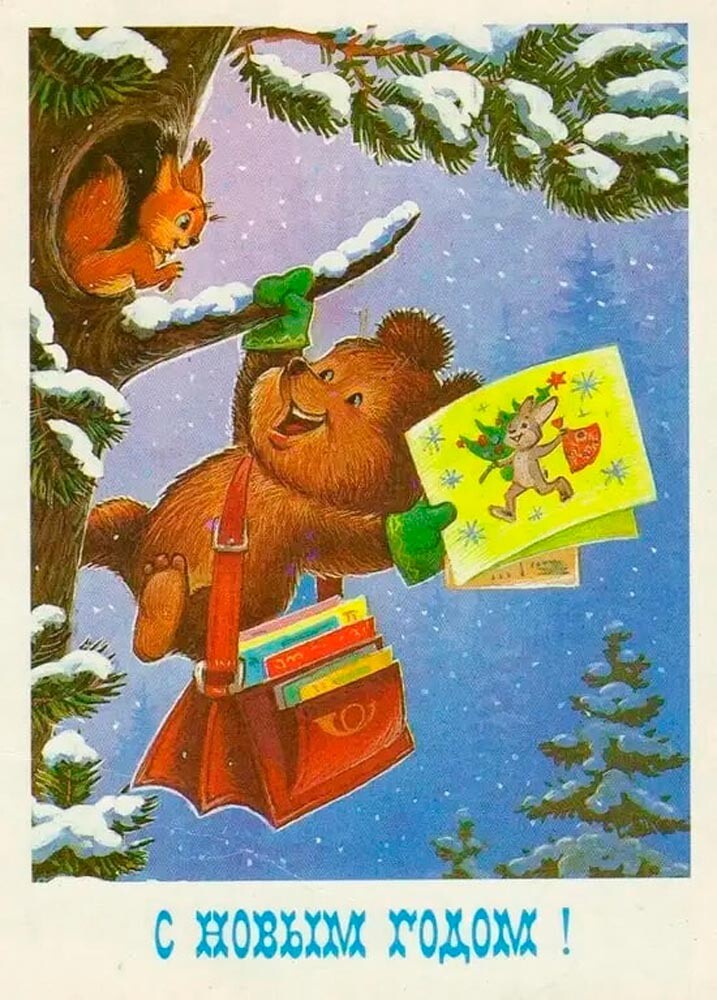In the image, a beautifully detailed, hand-drawn Christmas scene unfolds, capturing a whimsical moment between a bear and a squirrel. The bear, dressed only in green gloves, clings to a snowy evergreen tree branch. He carries an oversized red messenger bag overflowing with mail and postcards, some of which he holds in his right hand. The frontmost postcard depicts a rabbit carrying a Christmas tree and a sack of toys. The bear's cheerful expression mirrors the excitement of the squirrel peeking out from its nest in the tree trunk. Snowflakes fall gently in the dark, starry sky, blanketing the pine needles and branches. The scene is framed by an off-white, cream-colored border, with festive text at the bottom reading "Oblom Rao!" in blue letters, likely wishing Merry Christmas or Happy Holidays in another language. The background reveals glimpses of snow-covered, conical Christmas trees, further enhancing the holiday spirit of this colorful, animated cover, reminiscent of a children's book or a charming Christmas card.